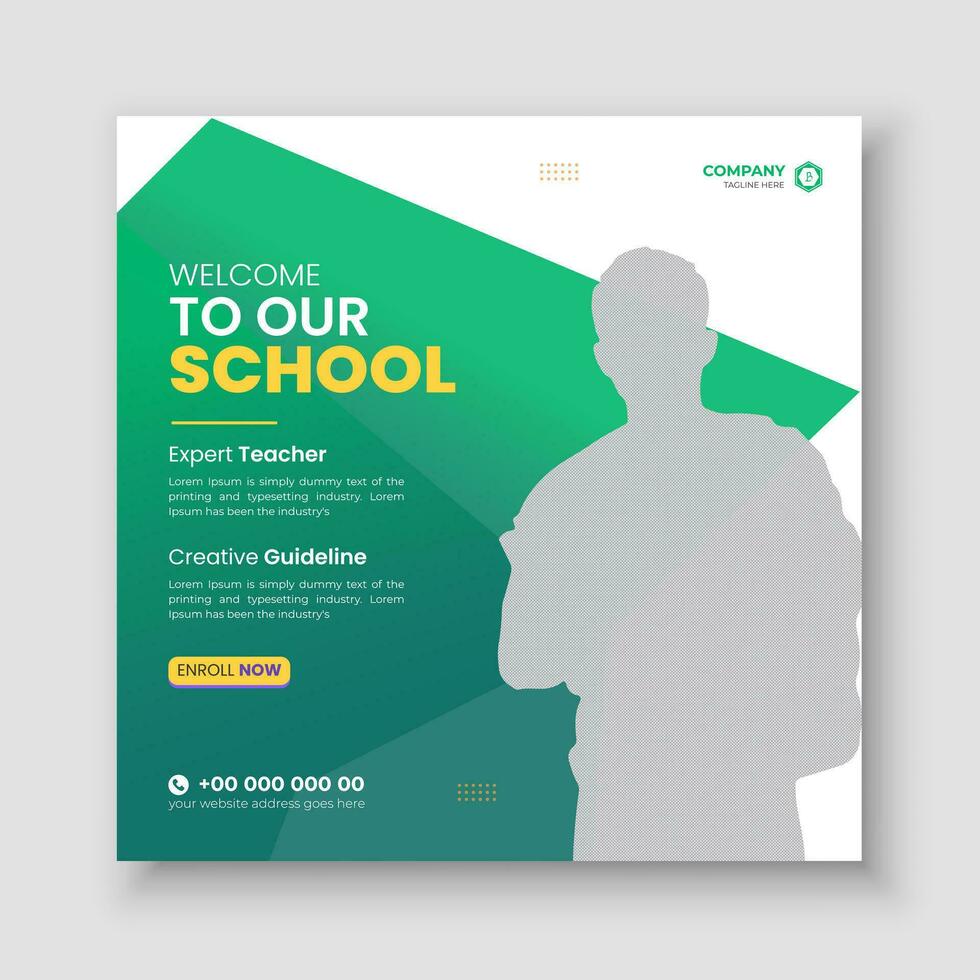This is a square-shaped advertisement featuring a white, green, and yellow color scheme with gray accents. The background is primarily green with various square and rectangular shapes. On the top left, bold text reads, "Welcome to Our School. Expert Teachers." Adjacent to it on the top right, a placeholder text states, "Company Tagline Here." 

Central to the design is the phrase, "Lorem Ipsum is simply dummy text of the printing and typesetting industry," serving as a filler for future content. Below this, there's a prompt to "Enroll Now," with designated spaces for a phone number and a website address at the bottom. 

On the right side of the ad, there's a gray silhouette of a younger man with a very short haircut. He appears to be carrying a couple of books and possibly a backpack, adding a dynamic and academic feel to the design.